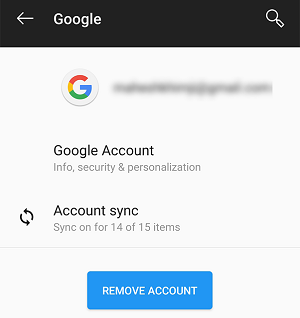In this detailed screenshot set against a clean white background, the header is solid black with crisp white text that reads "Google." On the left side of this header, there is a white left-pointing arrow. A white magnifying glass icon, representing search functionality, is also visible within the header.

Directly beneath the header, a small, round, white circle with a very slight gray border features the Google "G" icon. Adjacent to this icon on the right is a line of black text that has been deliberately blurred to obscure its content. Underneath this line of text, there are three sections labeled "Google Account," "Info," "Security," and "Personalization" in small, gray text, all aligned in one line.

Further down, in prominent black text, the words "Account Sync" are displayed. To the left of this text is an icon showing two arrows forming a circular shape, representative of the sync functionality. Below "Account Sync," it states "Sync on for 14 of 15 items" in a smaller font.

Towards the bottom of the screenshot, there is a blue action button labeled "Remove Account," ready to be tapped if the user wishes to disassociate the account.